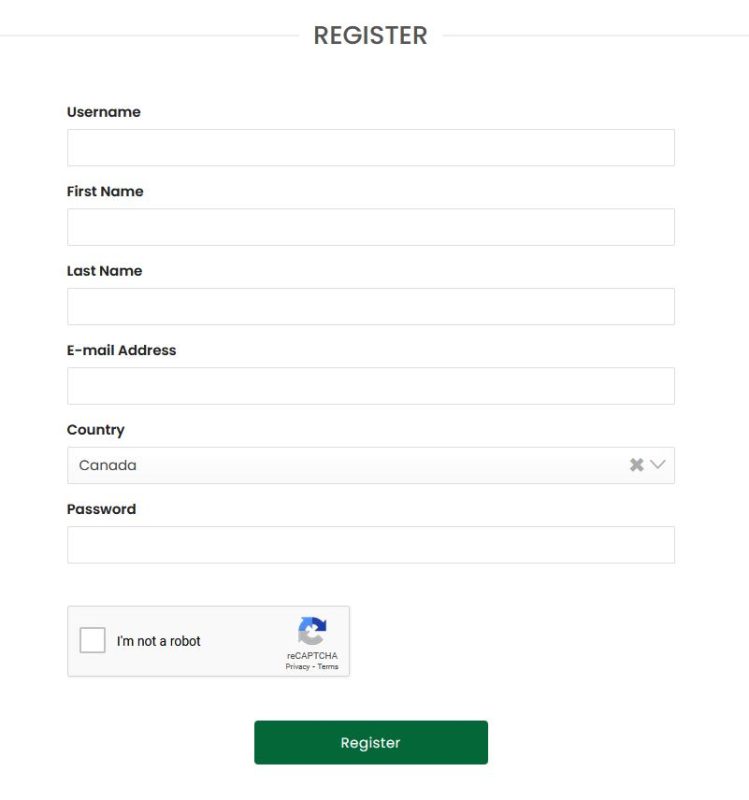The image depicts a minimalist yet functional web registration form, suitable for various devices such as smartphones, laptops, and tablets. The form opens with the heading "Register" at the top in dark grey letters, signaling its purpose. Below this heading, on the left-hand side, there is a series of fields awaiting user input, each labeled in bold black text.

The first field is labeled "Username" and is currently empty, inviting the user to enter their desired username. Moving downwards, the form continues with fields for "First Name" and "Last Name," both also in bold black text and presently blank. Below these are fields for "Email Address" and "Password," similarly styled and empty.

One field among them differs slightly—the "Country" field. It is pre-filled with "Canada," indicating the user's country. 

At the bottom of the form, but slightly offset to the left, there is a CAPTCHA verification section. This lightly grey-off white rectangle features a white checkbox on the left, next to the black text that reads, "I am not a robot." To its right, a circular arrow icon, partially blue and grey, is accompanied by the text "reCAPTCHA." Below this icon, in smaller print, are the terms "Privacy" and "Terms," providing a complete and secure registration experience.

This form exemplifies simplicity and clarity, ensuring users can effortlessly input their information and complete the registration process.